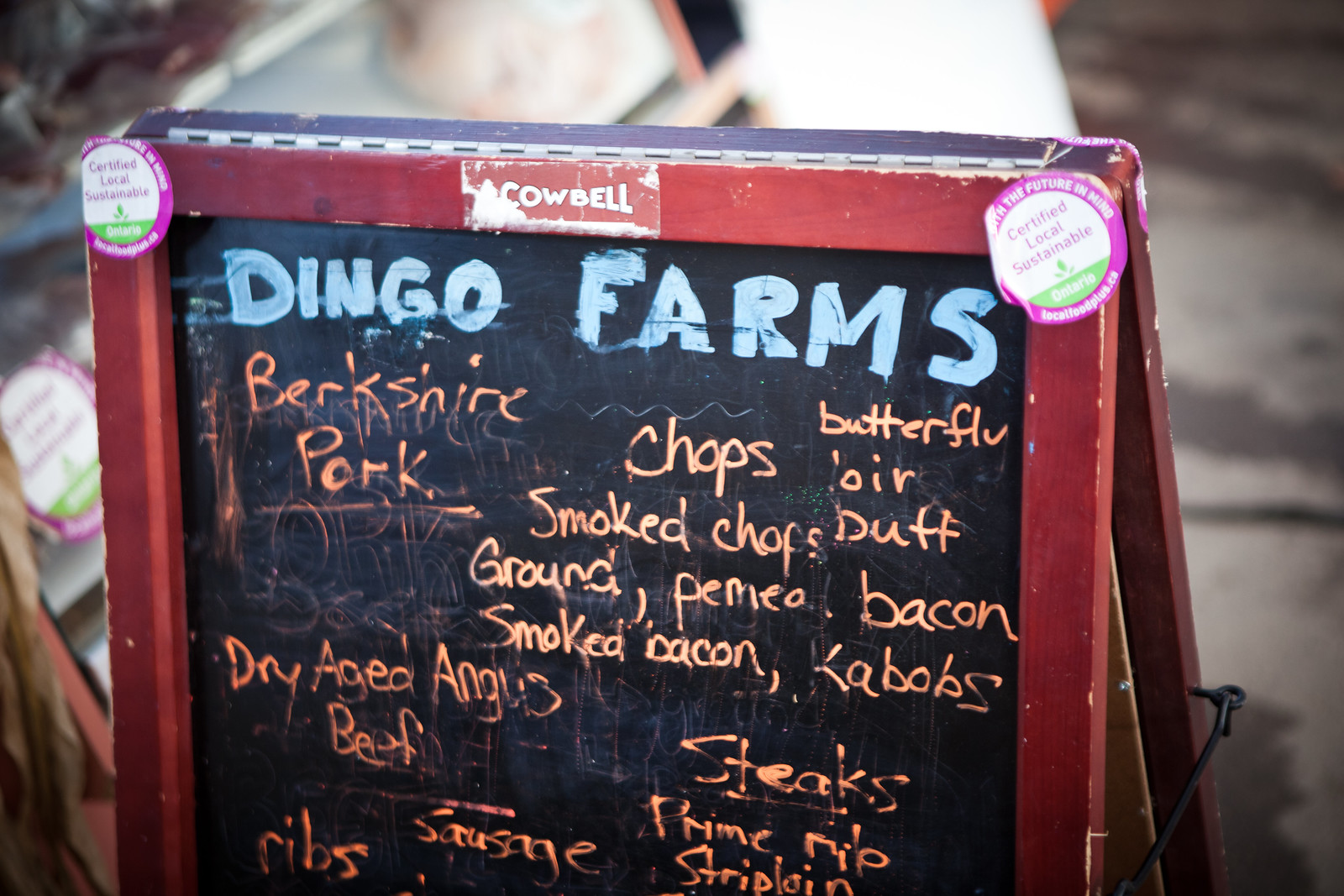The image depicts the upper half of a wooden A-frame sandwich board standing on a sidewalk. The board's frame is painted a reddish-brown color, and it has a black chalkboard inset that prominently displays the name "Dingo Farms" in blue chalk at the top. Below this, a list of farm products is written in various shades of orange and brown chalk, including Berkshire Pork items such as chops, smoked chops, ground pork, and bacon, as well as Dry-Aged Angus Beef products like steaks, prime ribs, and strip loin. There are also mentions of more specific items such as kebabs and smoked bacon. The details continue with sausages and ribs, although some words are partially obscured. In the upper left and right corners, there are stickers with white backgrounds and pink borders, which state "Certified Local Sustainable." The background of the image is blurred, making it difficult to discern the specific shop or surroundings, though a sidewalk and possibly a wet road can be seen.